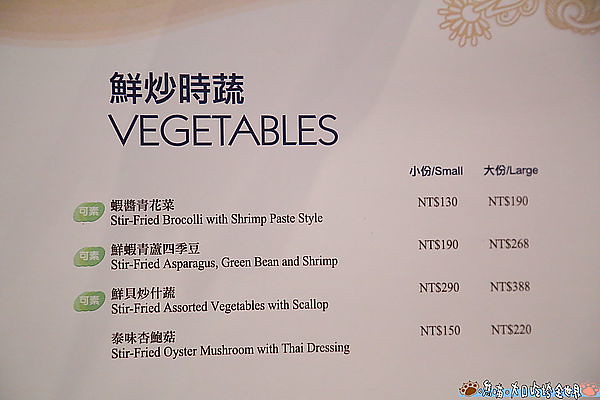The image shows a section of a menu with a clean, white background accented by a slight yellow curve in the top left corner and stylized yellow floral patterns on the right. Each dish name is listed first in Asian characters, followed by its English translation. This section, labeled "Vegetables," features dishes with varying prices for small and large portions. The menu includes:

1. Stir-Fried Broccoli with Shrimp Paste Style (NT $130 for small, NT $190 for large).
2. Stir-Fried Asparagus, Green Bean, and Shrimp (NT $190 for small, NT $268 for large).
3. Stir-Fried Assorted Vegetables with Scallop (NT $290 for small, NT $388 for large).
4. Stir-Fried Oyster Mushroom with Thai Dressing (NT $150 for small, NT $220 for large).

Decorative elements include a light brown, scribble-like pattern in the upper right corner and cartoony paw prints near some Asian characters in the bottom right.